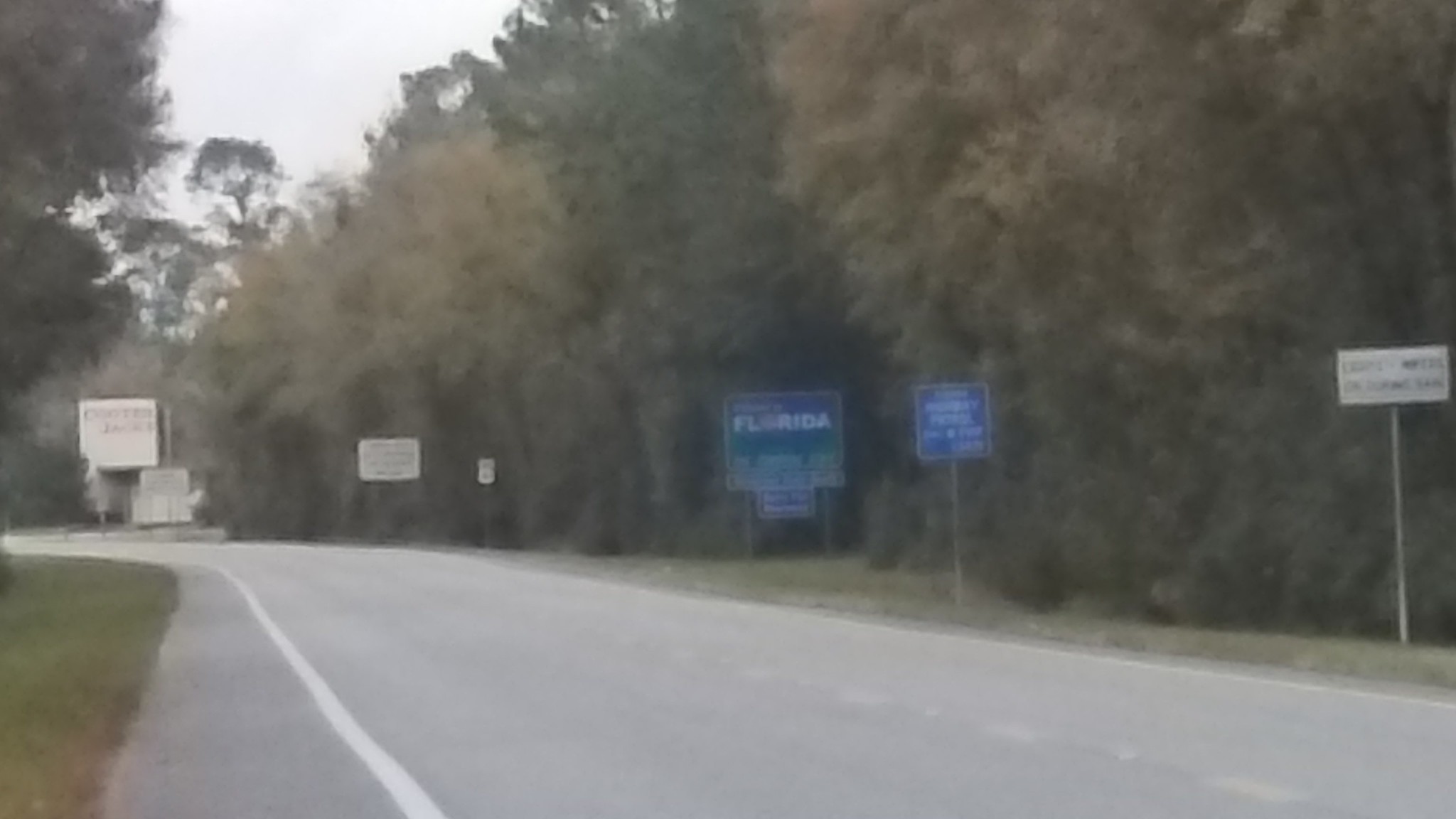This is a horizontally rectangular and somewhat blurry image, depicting a two-lane asphalt road seen from the left-hand shoulder. The image's resolution is grainy, adding to the overall haziness. The road features a white dotted line down the center and solid white lines along the edges. The road continues straight for approximately 20 yards before sharply curving to the left. On the right side of the road, there are five or six traffic signs with a mix of blue and white colors, one of which clearly reads "Florida." Beyond these signs, a dense wall of tall, bushy trees, some with leaves turning yellow, lines the right shoulder. The overall palette of the image appears muted due to its blurred quality.